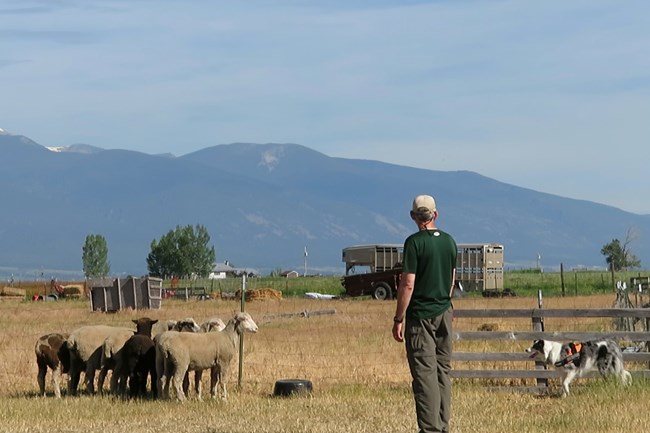In this detailed photograph of a farm, the central figure is a man standing with his back to the camera, wearing gray pants, a green shirt, and a white to off-white baseball cap. He appears to be gazing thoughtfully at the imposing mountain range in the background, where a touch of snow caps the tallest peaks. To his left, a small group of sheep clusters near the edge of a wired fence, while to his right, a black and white herding dog, donning a small vest, intently watches the sheep. The farm scene includes scattered trailers behind the man, assorted junk strewn around the brown grassy field, and sparse greenery with only a few trees dotting the landscape. Visible in the distance, there are green patches of grass, hay bales, and utility poles, adding further depth to the rustic setting.